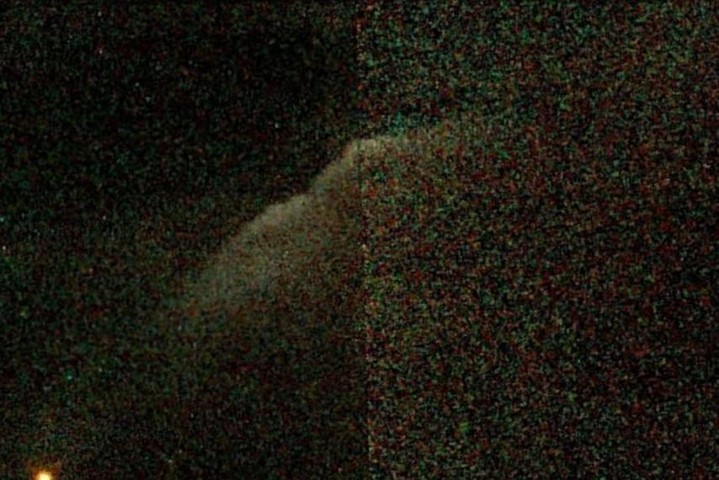This is an image set against a black background, bisected vertically by a line composed of minuscule, multicolored dots. On the right side, these dots—red, blue, yellow, brown, green, and other hues—are densely packed, with just a hint of the black background peeking through between them. Toward the center of the image, a muted, blurred white circle emerges, seemingly adorned with two gray eyes. Extending from this central figure are two large white wings, most discernible on the left side. The left side itself is predominantly black, featuring fewer and less prominent colored dots compared to the right. Additionally, in the lower left-hand corner, there is a notably larger yellow dot, resembling a sun or star, standing out against the multitude of smaller specks of light scattered across the image. The overall effect is reminiscent of an owl flying directly towards the viewer, surrounded by a cosmic backdrop of colorful specks and dots.